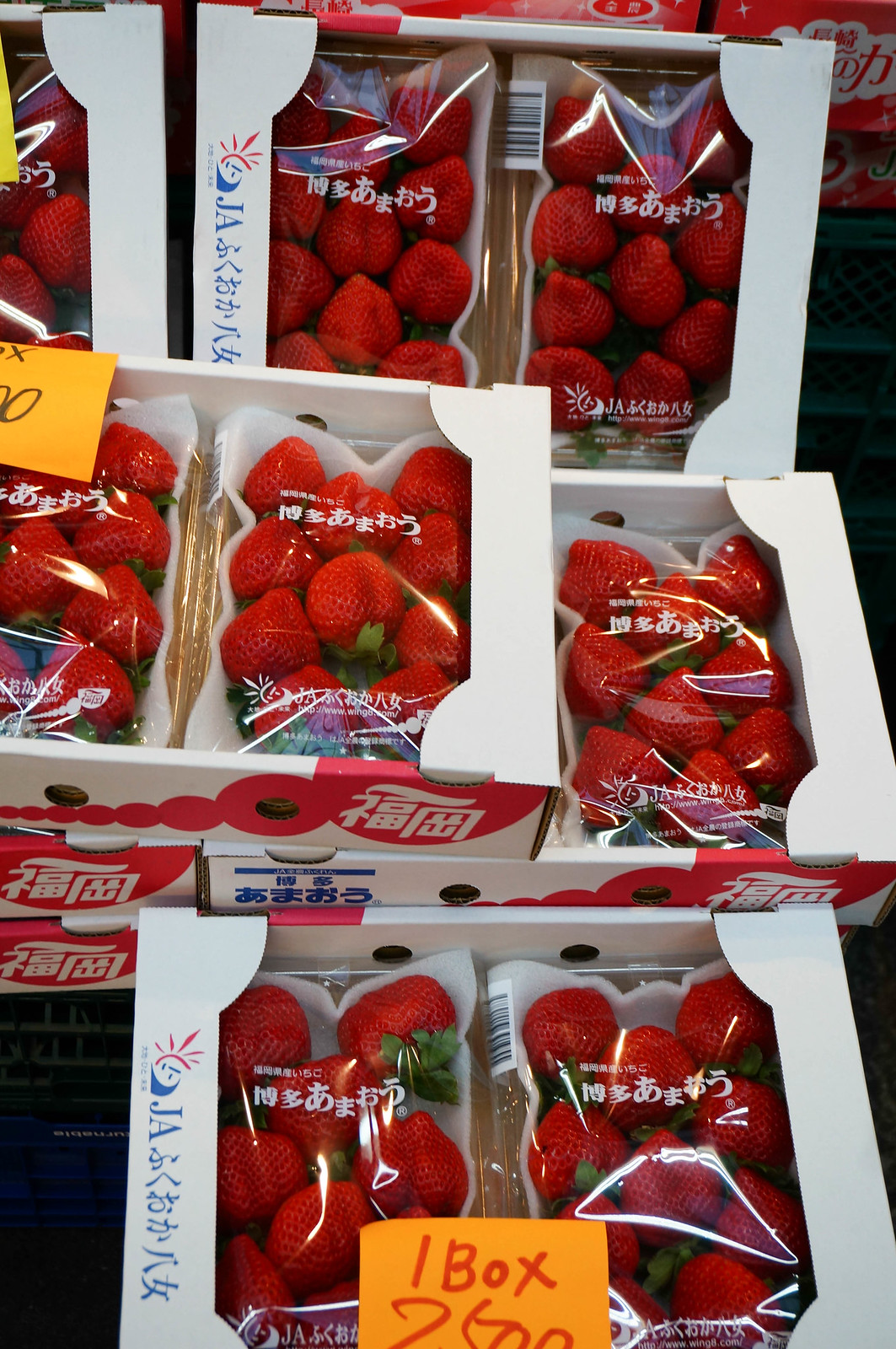The photograph showcases a vibrant display of fresh, red strawberries, neatly arranged in clear plastic-wrapped packaging, stored within small cardboard crates. Displayed prominently, there are around nine crates, stacked in an orderly manner, with some crates more forward-facing within the image. Each crate is labeled with an orange sticky note featuring red lettering, although the majority of the text is in an unidentifiable Asian script—likely either Japanese, Mandarin, or Korean—with the only legible English text reading "one box." The strawberries appear very healthy and ripe, their bright red color standing out clearly through the transparent packaging. Additionally, the setting could possibly be an indoor or outdoor store display.